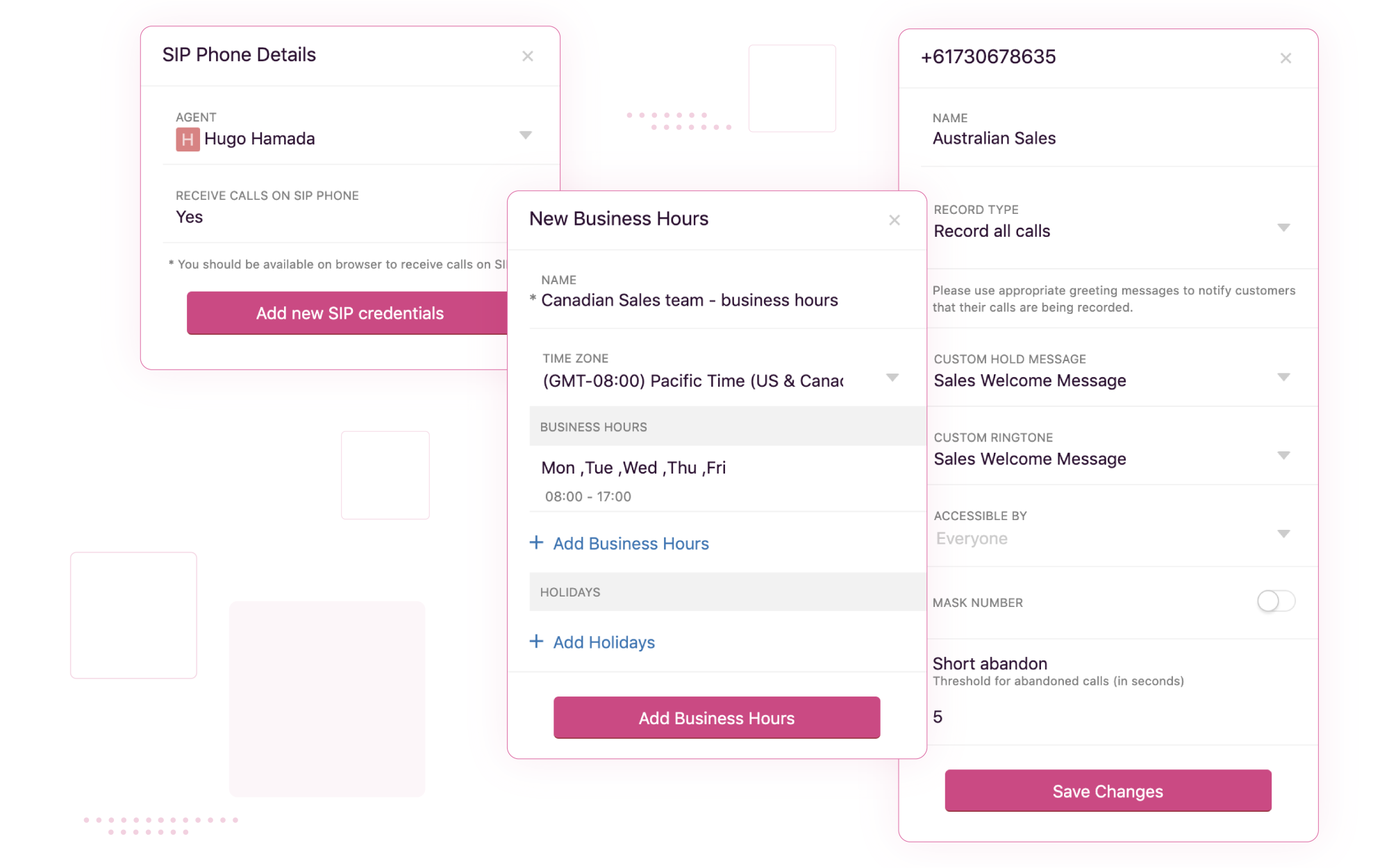The image depicts a section of an application interface with three distinct boxes, each framed by a thin red border and containing black text.

On the left, the smaller box is titled "SIP Phone Details." It features a close button (denoted by an 'X') in the upper right-hand corner. Below the title, there is a field labeled "Name," followed by a setting indicating the option to receive calls, which is marked as "Yes." At the bottom of this box is a prominent red button labeled "Add New SIP Credentials."

The central, larger box is titled "New Business Hours." It provides details for the "Canadian Sales Team Business Hours," including the applicable time zone and dates. At the bottom of this box, there is a red button labeled "Add Business Hours."

The final box on the right, which is also large, displays a phone number at the top, followed by a field labeled "Name." Below that is a section for "Record Type," indicating an option to record all calls. At the bottom of this box is a red button labeled "Save Changes."

Each box is clearly outlined and structured, facilitating ease of use and navigation for the user.